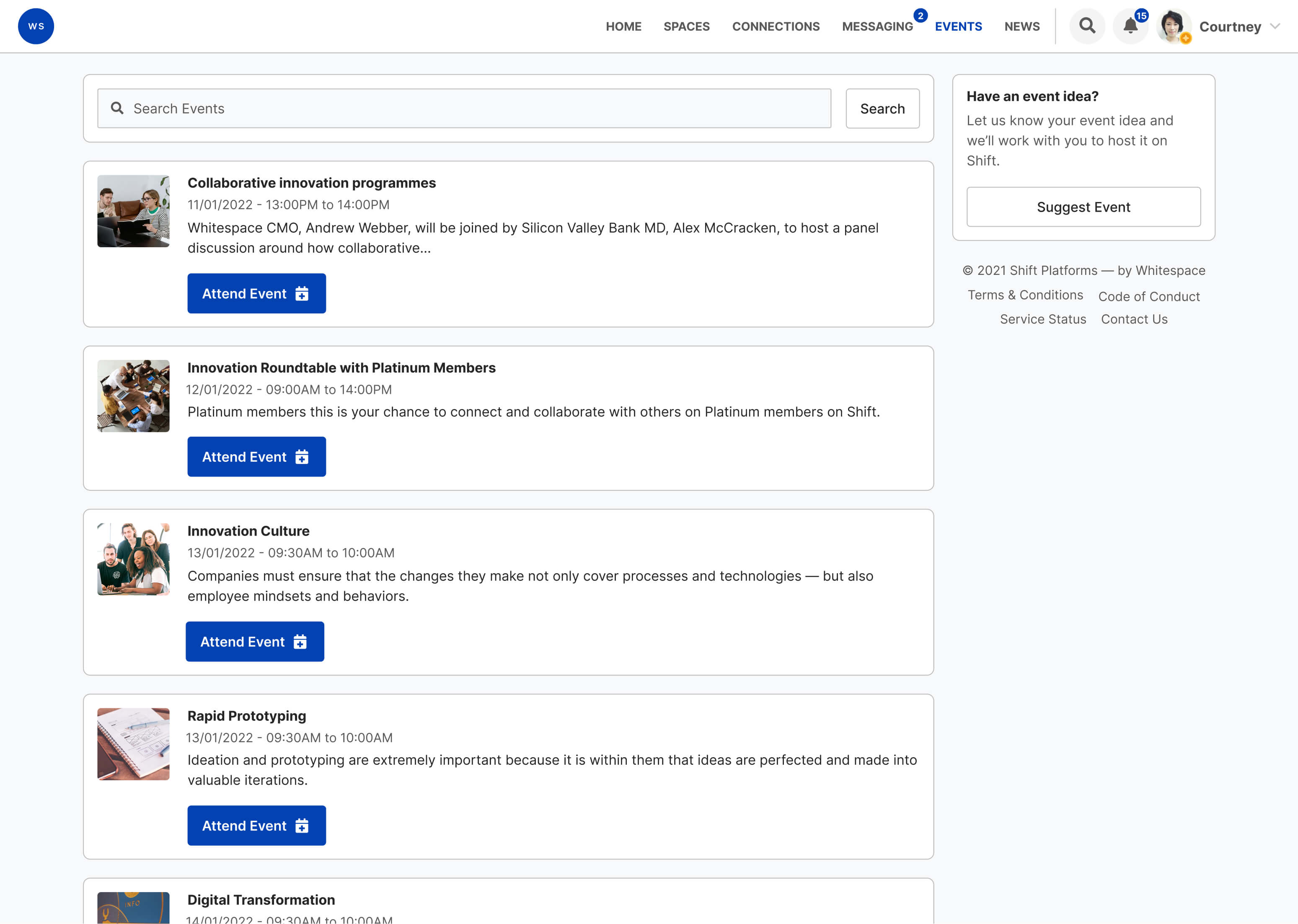The website features a blue circular button in the upper left-hand corner with the letters "WS" inscribed on it. Moving horizontally across the page, a navigation bar becomes visible, listing options such as Home, Spaces, Connections, Messaging, Events, and News. A blue dot above the Messaging option indicates there are two new messages. 

Further along, there are icons for searching and notifications, with the latter showing 15 alerts. A profile picture labeled "Courtney" appears toward the top, accompanied by a drop-down menu, suggesting multiple profiles are in use. Below this, a search bar labeled "Search Events" and a corresponding search button are prominently displayed.

Beneath the search bar, a series of events are listed, each accompanied by a thumbnail image. Each event has a blue rectangular "Attend Event" button beneath it, written in white text. The events include:
1. Collaborative Innovation Programs on November 1st, 2022.
2. Innovation Roundtable with Platinum Members.
3. Innovation Culture.
4. Rapid Prototyping.
5. Off the Page Digital Transformation.

To the right of these listings, there is an option for users to suggest their own event ideas.